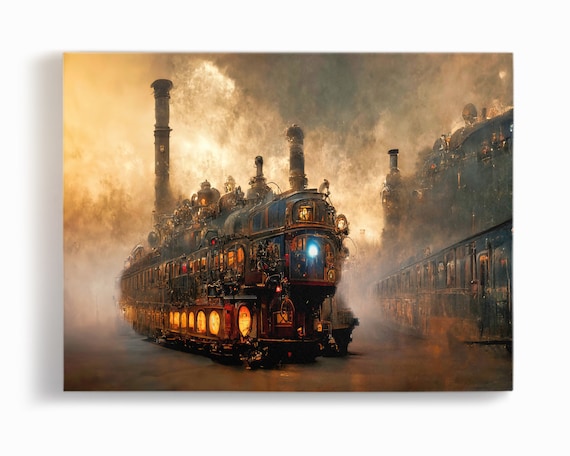The image is a multi-colored, detailed artistic piece that could be made with ink, paint, or digital mediums. It is square, with a very faint off-white border surrounding it, and an evident shadow on the left side where it meets the background. The central focus of the art is an ornate, old-fashioned locomotive, depicted with a moody and smoky ambiance, transitioning from orange to white in the center, to black on the right. The locomotive features blue lights on the front and reddish-orange lights along its side, with lit-up windows and gold circles positioned above the wheels. There are plumes of steam throughout, adding to the smoky atmosphere. Additionally, the painting includes what appear to be various structures or buildings with smokestacks in the background and train cars located in the lower and upper right-hand corners. The overall scene evokes a sense of movement and mystery, capturing the essence of an old train journey through an industrial landscape.